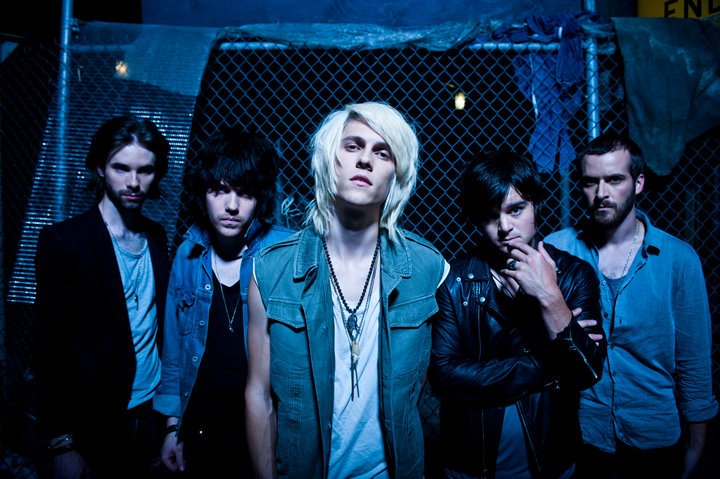The photograph depicts a group of five young men in their mid-twenties, likely a rock or punk band, standing in front of a crumpled, tarp-covered chain link fence in a dimly lit environment. The focus is on the man in the middle, who is white with thick, almost shoulder-length blonde hair. He wears a blue jean vest over a very short-sleeved white t-shirt, accessorized with a chain and baubles. Flanking him are four other men, all with serious, intense expressions and medium-length dark hair. To his immediate left is a shorter man in a black leather jacket over a blue shirt, and to the far left, a bearded man with dark hair, wearing a blue jean shirt and a tank top underneath, along with a chain necklace and dark pants. On his right stands another man with nearly face-covering black bangs, dressed in a black shirt, chain, and blue jean jacket, adorned with a watch band. At the far right is another bearded man with long brown hair, almost shoulder length, clad in a black jacket and a blue tank top beneath, also wearing a chain and black pants. Overall, the photo has a dark, brooding atmosphere with heavy light reflections on their faces, highlighting their serious expressions.